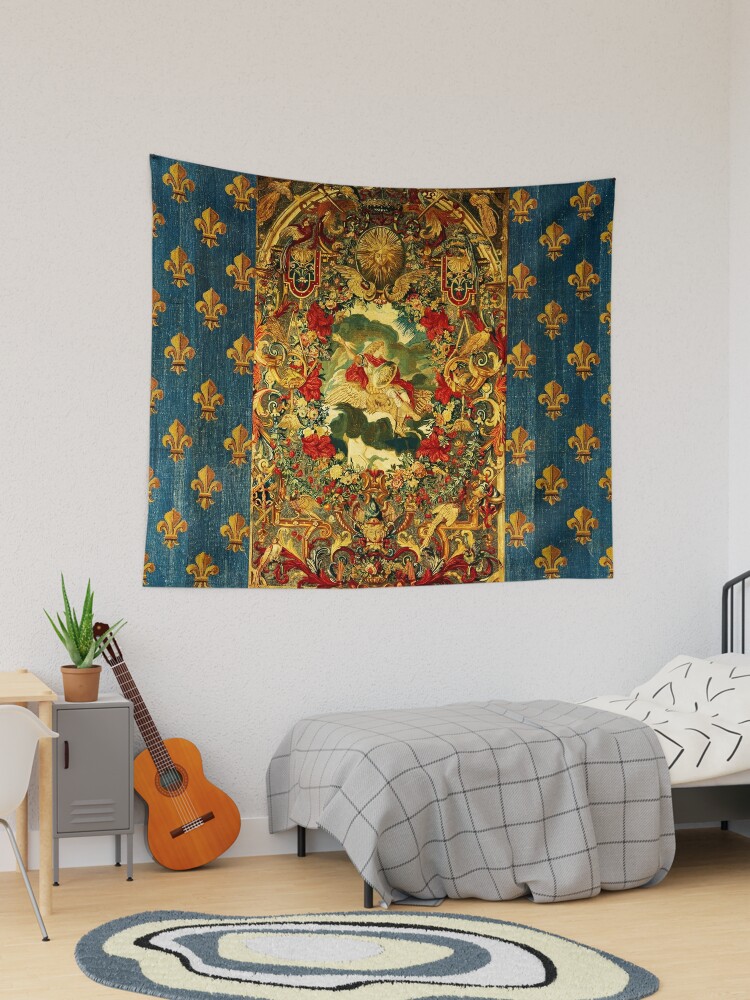The photograph captures a cozy bedroom with a light pine wooden floor, adorned with a distinctive circular rug featuring wavy, uneven rings in gray, yellow, black, and white. The focal point of the room is an ornate tapestry hanging on the wall, showcasing an intricate design, framed by blue panels adorned with fleur-de-lis on either side. The centerpiece of the tapestry includes detailed depictions of red, gold, and green figures, possibly including angels.

To the right of the image, there is a twin bed with a black metal frame, dressed with a gray checkered bedspread and white sheets bearing an arrow pattern. Leaning against a small gray metal cabinet beside the bed is a guitar. This cabinet also supports a spiky potted plant, likely a succulent or cactus.

A small corner of a wooden desk, paired with a plastic chair on metal legs, is visible next to the cabinet. The overall arrangement and decor give the impression of a simple yet personalized space, possibly belonging to a teen or a college student.